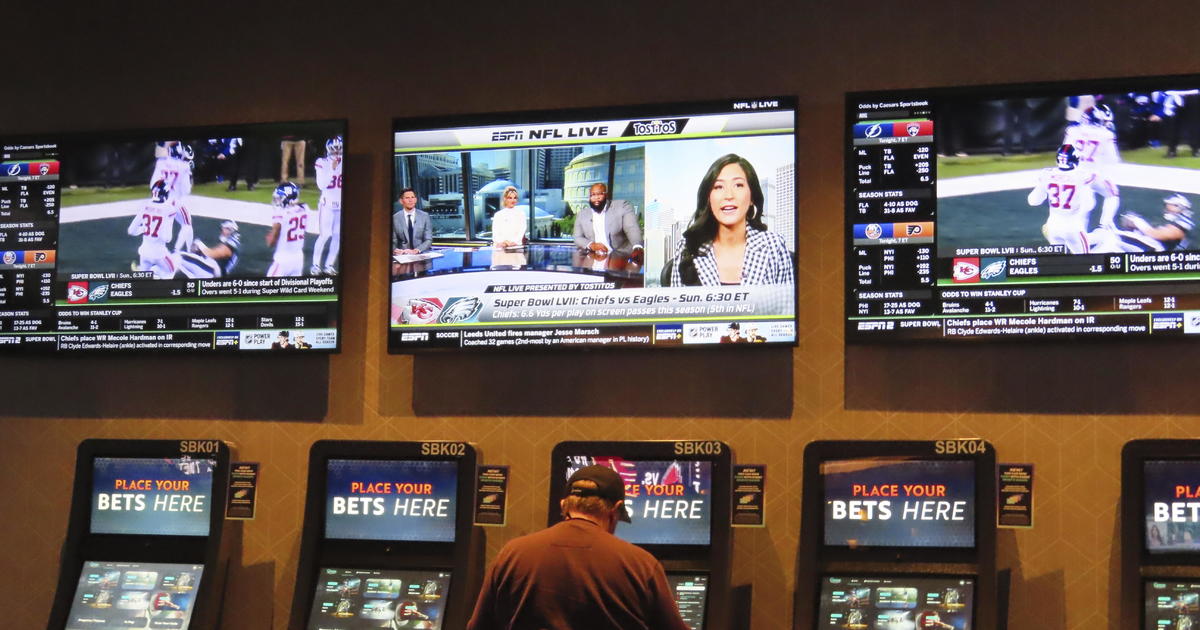The image features a dark tan wall at a casino sports betting area. Prominently, there are three TV screens mounted on the wall, each displaying different sports content. The left and right screens feature football games, while the center screen shows an ESPN talk show with information about an upcoming Chiefs vs. Eagles Super Bowl. Below the TVs, five black betting terminals are lined up, each with the prompt "place your bets here." The terminals are labeled SBK01 to SBK05, but only the first four numbers are visible. At one of the terminals, a man in a ball cap and red shirt is seen from about halfway up his torso, engaged in placing a bet. The ambiance is somewhat dim, typical of a casino environment.